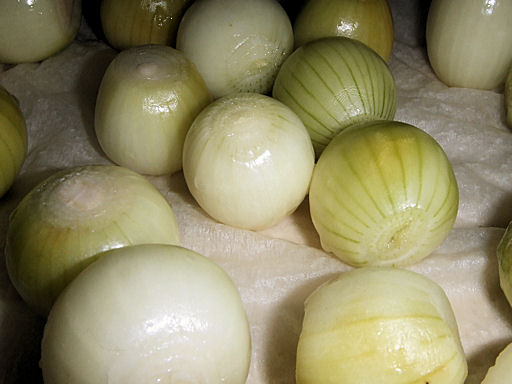This image is a close-up of approximately 15 peeled onions, meticulously arranged on a white cloth, possibly a paper towel. The onions are predominantly white, but a few exhibit green hues and darker green stripes running horizontally or vertically. Some also show subtle yellowish-brown tints, indicating remnants of their outer layers that might not have been completely removed. Each onion has its ends cut off, giving them a uniform, shiny appearance. The composition is centered around a cluster of about five onions, with the rest dispersed around this central group. The indoor lighting is evidenced by the visible light source reflecting off the onions and the faint shadows cast around them.